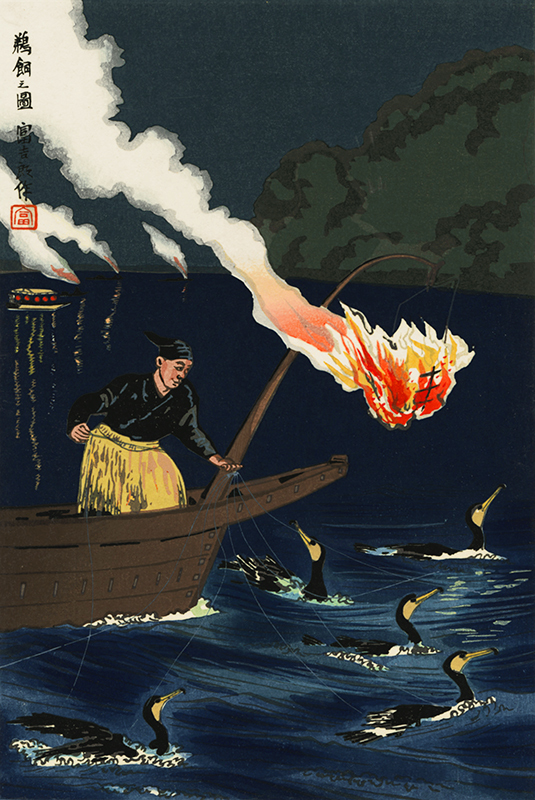The image is a detailed painting of a nighttime lake scene in an old Asian style. The scene primarily uses shades of blue, with the lake rendered in a darker blue and highlighted by white streaks to depict waves and current. Above the lake, the night sky is a different shade of blue, with a green hill and trees on the right-hand side.

In the foreground, near the bottom left, is a brown, wide-front wooden boat. In this boat stands a man wearing a black long-sleeved kimono and wide, baggy yellow pants, along with a black hat. Suspended from a wooden pole at the front of the boat is a burning lamp, casting light onto the water. 

The man is fishing using five black cormorants, which are tethered with strings around their necks that he holds as he leans over the edge of the boat. The water beneath shows the ducks—or cormorants—with their yellow bills and heads. Fireballs or flaming arrows appear to fall from the sky, creating smoke and illuminating the scene.

In the upper left corner of the painting, Chinese text is inscribed, adding to the cultural atmosphere. The colors prominent in this image include various shades of blue, red, yellow, black, navy, white, green, and brown.